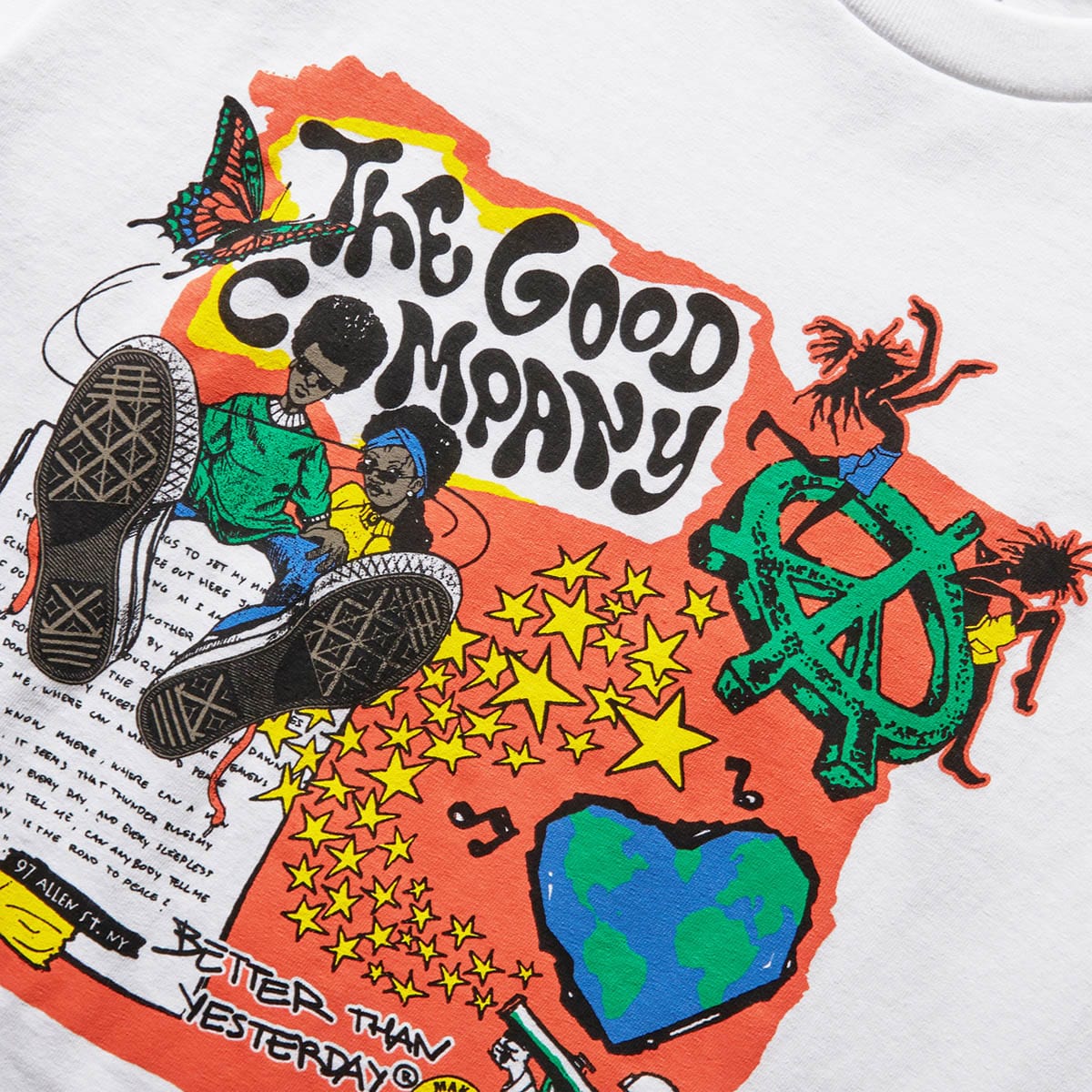The image is a close-up of a white t-shirt featuring an intricate and colorful graphic design. The design includes a red background with the text "The Good Company" in bold black letters outlined in yellow, located in the top left corner. The 'O' in 'Company' is cleverly represented by the head of a man of African descent with a large black afro. He is wearing sunglasses and a green long-sleeve shirt with blue jeans. His pose is dynamic, as if he is standing above the viewer, revealing the bottoms of his shoes.

Next to him is a black woman adorned with a blue bandana and sunglasses, wearing a yellow sweater. To the right of them, stars appear to be shooting out from a bazooka positioned below. Above, a heart-shaped Earth and a peace symbol with people dancing around it add to the vibrant, hippie-inspired theme. Beside the word "The Good Company," a butterfly floats gracefully. Beneath the man is a lengthy letter, and to its right, the phrase "Better Than Yesterday" is scripted prominently.

Overall, the graphic is a lively and detailed representation of peace and unity, encapsulated on a t-shirt.